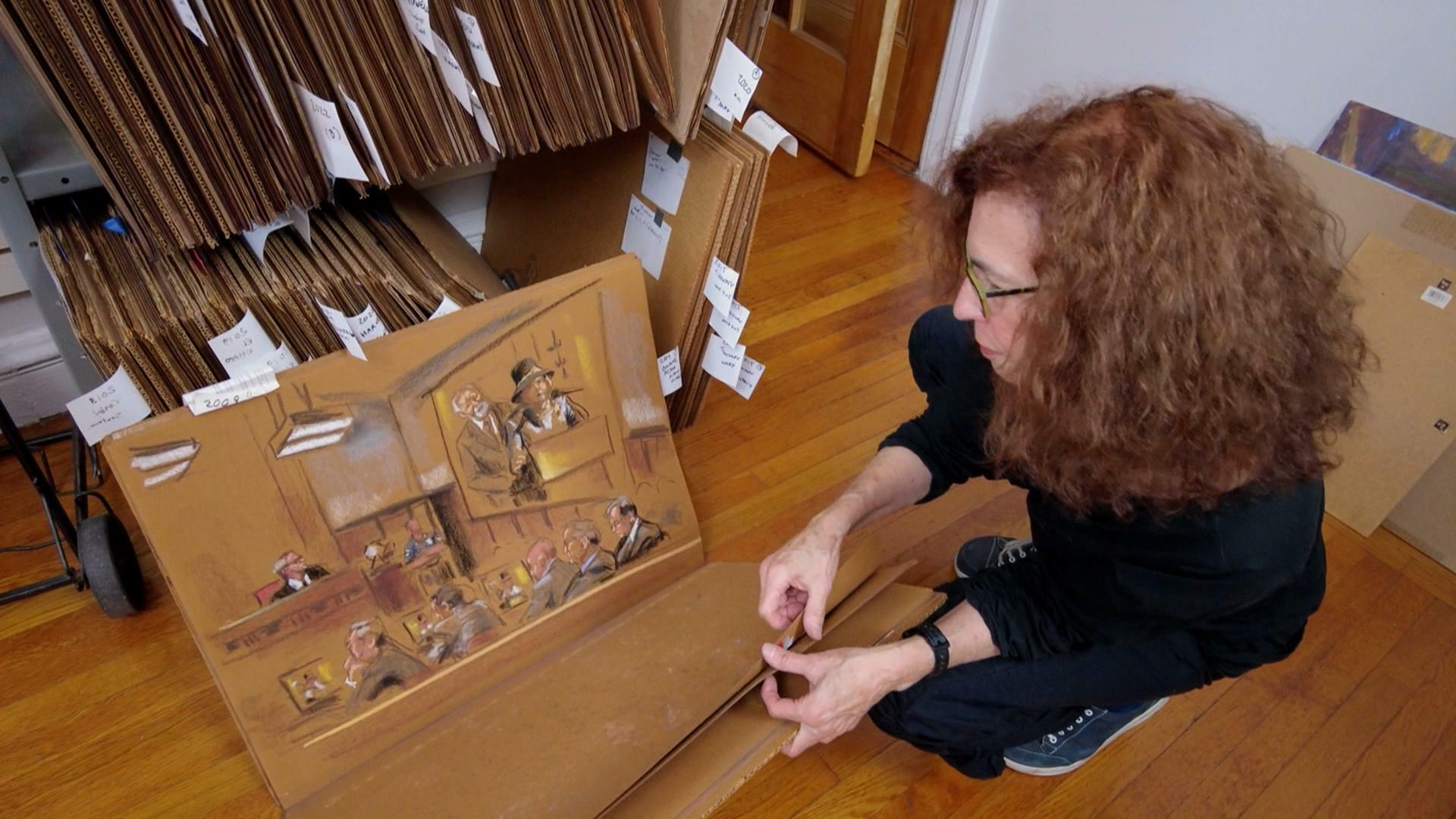The image shows a woman crouched down on a brown wooden floor, closely examining a court scene artwork resting on a cardboard piece. The artwork, primarily in brown tones, displays several figures including a judge and people watching a screen, all depicted on a tan or cardboard background. The woman, who appears to be in her late 40s to mid 50s, has frizzy, medium to long red hair and wears thin, black-framed glasses along with a long-sleeved black shirt and dark blue jeans. To her left is a silver metal shelf filled with numerous cardboard rectangles, each with white paper tags bearing black writing, though the text is difficult to read. Partially in the frame is a brown door with a white wall adjacent to it, providing additional context to the setting.